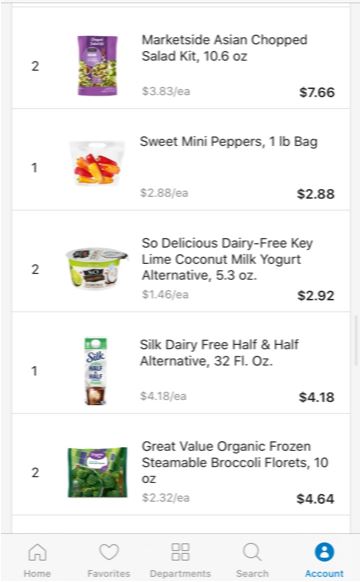Screenshot of a grocery ordering app displayed on a smartphone. The app interface features a menu at the bottom with five icons: Home, Favorites, Departments, Search, and Account. The shopping cart contains the following items: 

1. Two bags of Market Side Asian Chopped Salad Kit, each 10.6 ounces, priced at $7.66, shown in a purple bag.
2. One bag of Sweet Mini Peppers, weighing one pound, priced at $2.88, with yellow and red mini peppers visible.
3. Two containers of So Delicious Dairy-Free Key Lime Coconut Milk Yogurt Alternative, each 5.3 ounces, priced at $2.92, with one yogurt container displayed.
4. One carton of Silk Dairy-Free Half and Half Alternative, 32 fluid ounces, priced at $4.18, depicted with the Silk branding.
5. Two bags of Great Value Organic Frozen Steamable Broccoli Florets, each 10 ounces, priced at $4.64, shown in predominantly green packaging.

Each item includes an image for easy identification.